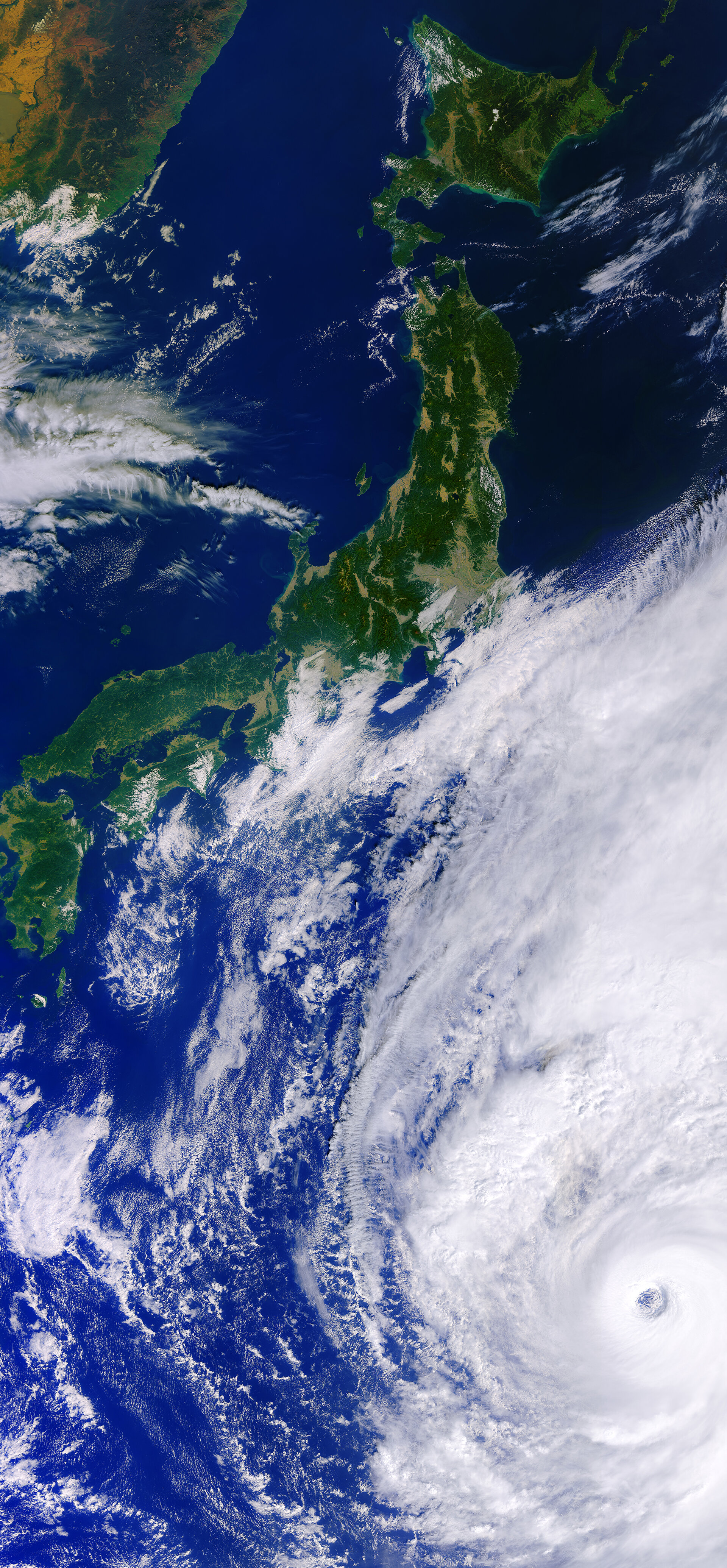The image is a narrow, vertical, rectangular photograph of planet Earth, likely taken from a satellite or low orbit. It prominently features the lush green landscape of an island or peninsula, potentially the islands of Japan, situated to the upper side of the image, with hints of additional landmasses such as parts of China visible in the upper left corner. Surrounding the land is a vast expanse of dark blue ocean. Dominating the lower right portion of the image is a partially visible, massive cyclone or tornado. The storm appears as swirling, thick, white clouds forming the classic spiral shape, with a distinct eye at its center, partially cut off by the edge of the image. This fierce weather system seems to be moving towards or possibly having already affected the visible landmasses.